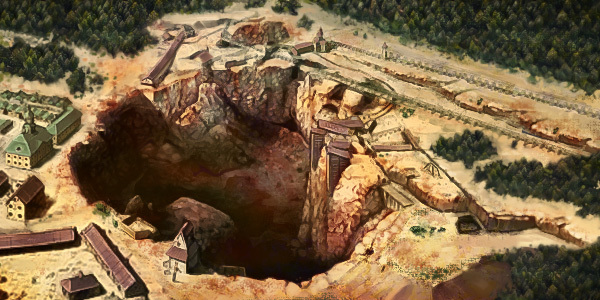This image, a vibrant and detailed painting, depicts a large quarry or sinkhole situated in a vast, arid desert region. Dominating the center of the image is the massive, gaping hole characterized by shadowed dark stones at its base and edged with gray and peach-colored rocks. Surrounding this monumental pit, particularly to its left, lies a small residential area adorned with two-story buildings indicative of the 18th century. These structures, some crowned with red or green pitched roofs, appear almost miniature in the presence of the colossal hole. In the right portion of the image, railways and industrial equipment suggest mining activity, possibly utilized for transporting extracted materials. The light tan ground contrasts with the lush, green forest that frames the top and extends partially down the right side, blending nature's vibrancy with the starkness of the quarry. Brown and red wooden scaffolding structures are constructed along the sides of the hole, hinting at efforts of excavation or stabilization, potentially following a disastrous event.